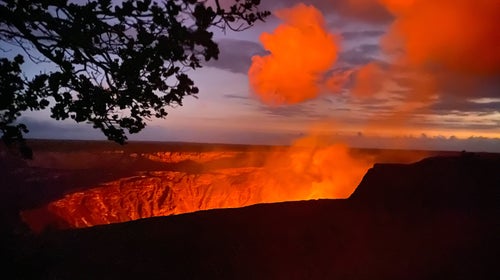The photograph captures a dramatic scene of a lava field at twilight. Dominating the foreground is a vast chasm that stretches from the bottom left towards the center right of the image, emitting an intense, fiery glow of bright orange and yellow, suggesting the presence of molten lava below. Plumes of steam and smoke rise from this chasm, blending into shadowy clouds that speckle the sky above. The foreground and surrounding rocky terrain are engulfed in deep shadows, providing stark contrast to the illuminated abyss. A silhouetted tree branch hangs down from the upper left corner, its dark form standing out against the colorful backdrop. The twilight sky showcases an array of hues, transitioning from pale blue to deep lavender and darker purples, with a trace of yellow lingering on the horizon, hinting that the sun has just set. The overall ambiance is one of intense heat and smoke, combined with the serene beauty of the fading daylight.